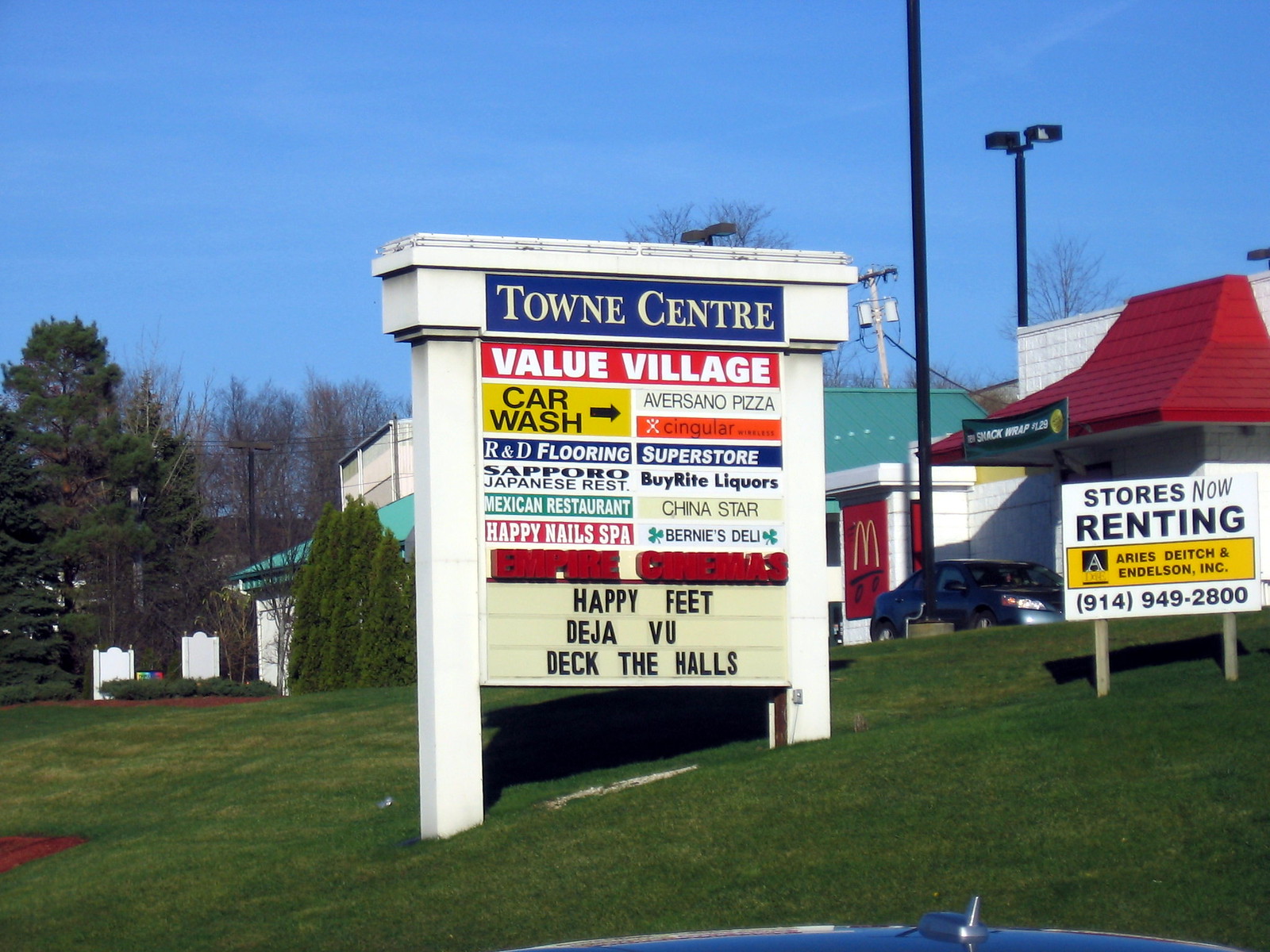This is a detailed photograph taken outside of the Town Centre shopping complex, featuring a prominent white sign with "Town Centre" in white capital letters on a blue background, mounted atop two white pillars. The sign sits on a grassy, slightly hilly terrain. Beneath the main sign, a series of smaller signs display the names of businesses within the complex, including Value Village, Car Wash, Aversano Pizza, Singular Telephone, R&D Flooring Superstore, Sapporo Japanese Restaurant, By Wright Richards, Mexican Restaurant, China Star, Happy Nail Spa, Bernie's Deli, and Empire Cinemas. The cinema marquee advertises current showings: Happy Feet, Deja Vu, and Deck the Halls. Below the main sign, there is a customizable message board with today's display reading "Happy Feet Deja Vu Deck the Halls." To the right of the sign, there is an estate agent's board indicating stores are available for rent, accompanied by a phone number. In the background, a McDonald's restaurant and several other buildings are visible, set against a clear blue sky, with both evergreen and leafless trees providing a natural backdrop.